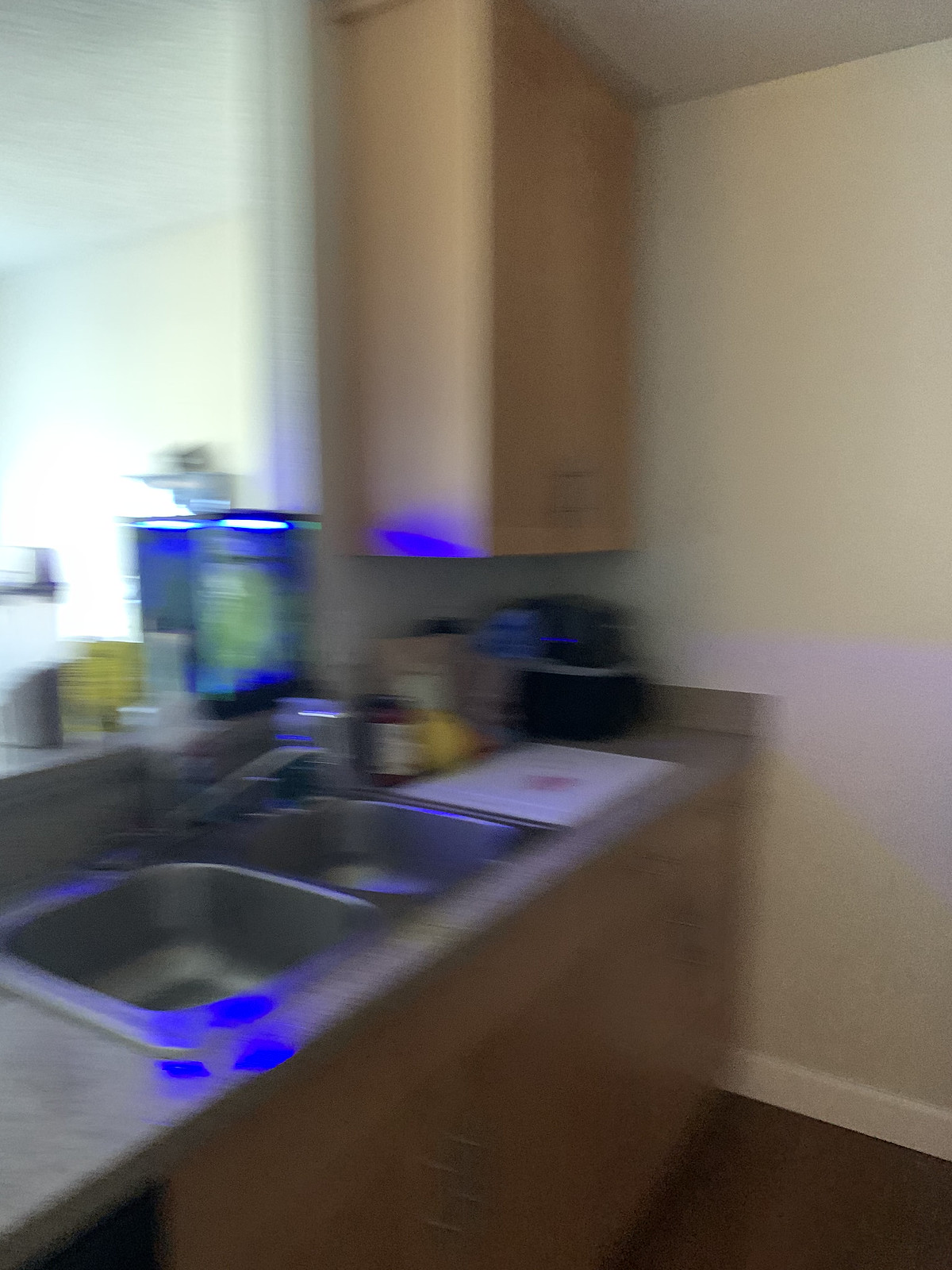This blurry photograph captures a kitchen interior roughly one and a half times taller than it is wide. The off-white, cream-colored wall frames the scene, with light brown wooden cabinetry lining the top right-hand corner. Central to the composition is a double-sided kitchen sink set within a grey marble countertop extending from the left edge of the image to about 80% across, intersecting with the far wall. The left side of the image hints at a window or another room providing additional light, illuminating parts of the kitchen. To the right of the sink lies a white plastic cutting board beside a jar and a yellow round object, while a black square container adds a stark contrast on the counter. Above the sink, we find a window, and behind it, a raised counter acting like a bar, which supports a rectangular aquarium emitting a faint blue glow. This glowing blue light interestingly casts patches of color onto the surrounding cabinets and surfaces, adding an unusual and captivating element to the somewhat blurry and indistinct scene.